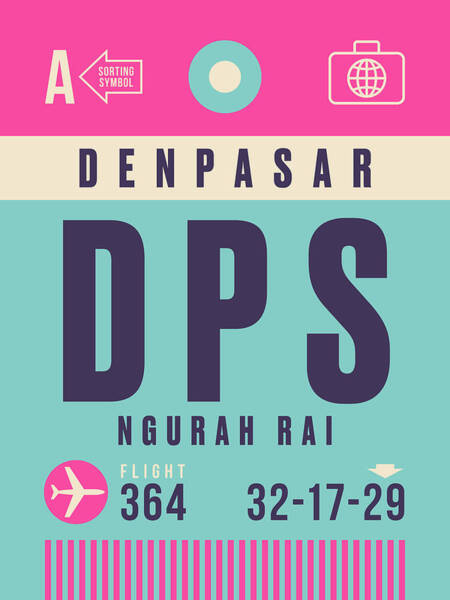This image is a vibrant, computer-generated poster with a structured layout featuring three distinct sections. The top 20% of the image has a bright pink background. On the left, a white letter "A" is accompanied by a left-pointing beige arrow that reads "sorting symbol." Next to it, a green circle with a white center sits in the middle, and a briefcase icon with a globe inside is on the right. The next section, underneath, is a small strip with a tan background displaying the word "DENPASAR" in black text. The majority of the image, about 75%, has a light green background with large dark blue letters "DPS" followed by smaller text "NGURAH RAI." Beneath this, a pink circle with a white airplane icon is shown, next to "flight 364." To the right, it lists "32-17-29," and the bottom of the image features a pink barcode-like pattern consisting of vertical lines running to the edge.